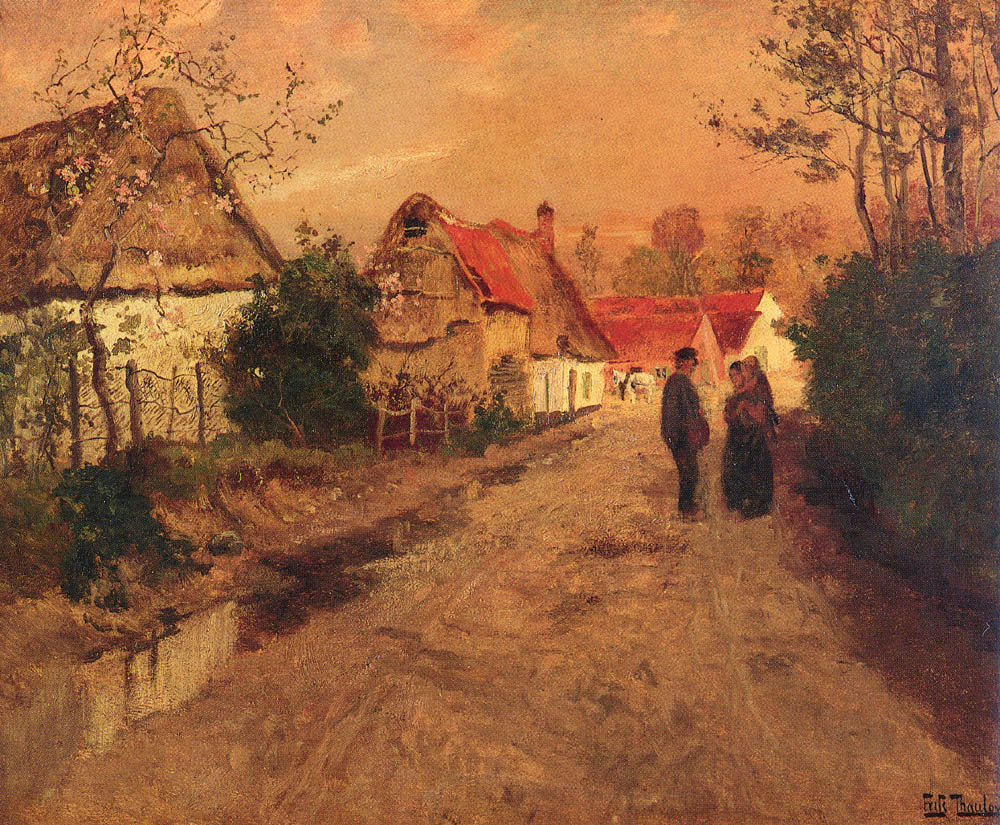This painting, done in an impressionistic style, vividly depicts an old, picturesque village from a dirt road vantage point. The scene features quaint, well-maintained cottages with steep roofs—some red, some brown, and a few thatched or hay-covered. The cottages' white siding and orderly appearance suggest they are centuries old. Dominating the warm, brownish-golden color scheme reminiscent of a sunset, the painting incorporates muted earth tones with occasional pops of red. 

In the foreground, a man in a black long-sleeve shirt and pants converses with two women; one woman cradles a baby in her arms, also dressed in dark, mostly black clothing. The sky above is dusky with a yellow-orange hue, adding to the serene atmosphere. The left side of the painting shows more cottages, likely enclosed by a small white picket or wooden fence, while the right side features a large green bush and smaller trees topped with pink blossoms. Tall trees with vibrant green foliage form the backdrop.

The dirt road, speckled with puddles, extends through the village, enhancing the rural charm. The overall composition, highlighted by earth tones and dominated by muted browns and greens, imbues the piece with a nostalgic, tranquil feel, capturing a moment in this timeless, old-world village.